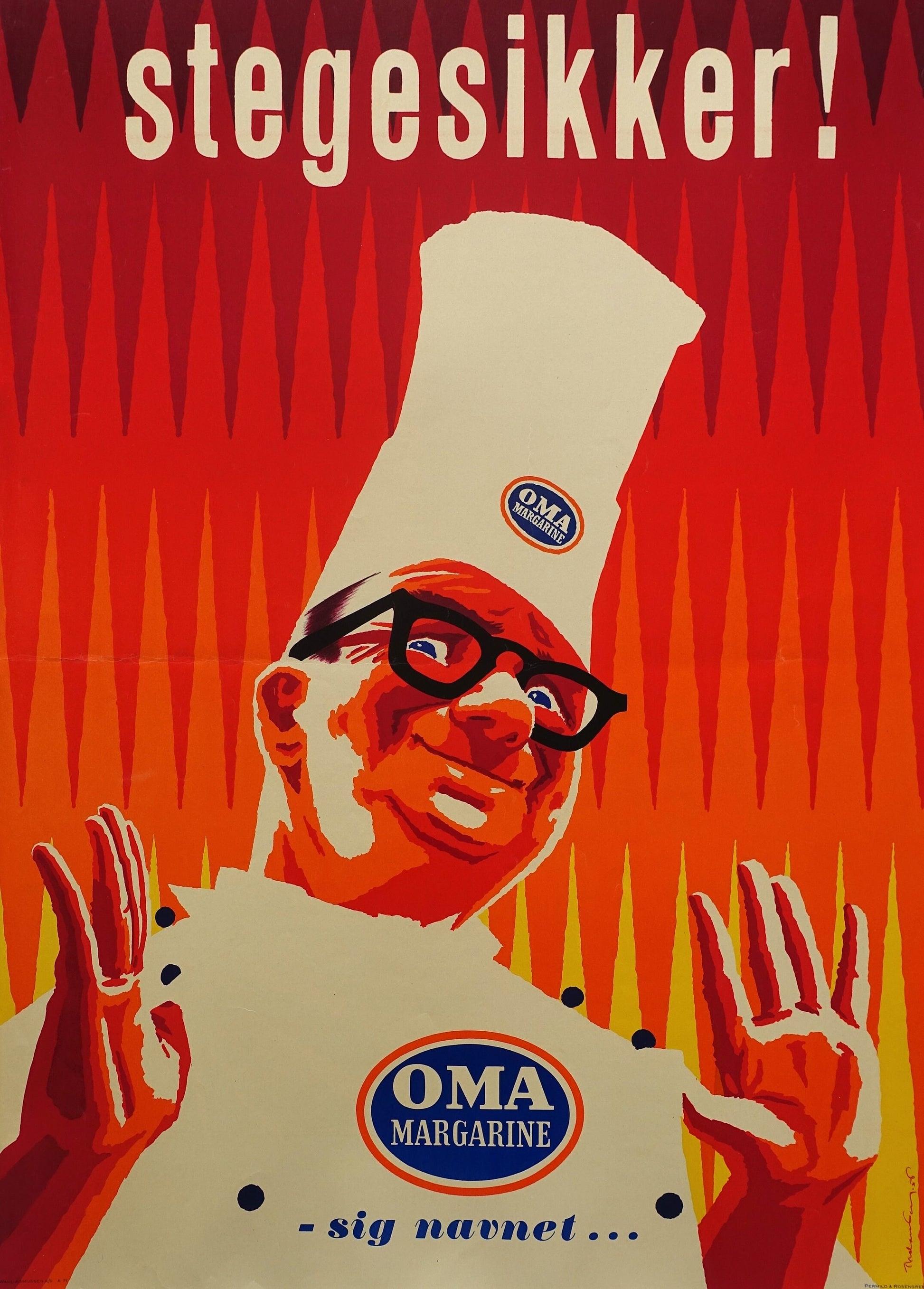The image appears to be an advertisement poster, characterized by a vibrant background composed of narrow, triangular lines with sharp tips, pointing both upwards and downwards. These triangular patterns transition in color from dark brown at the top, through various shades of red, orange, and then to yellow at the bottom. 

Centered at the very top of the poster, in bold white text, it reads "Stege Sikker!" Below this, the focal point is an image of a middle-aged man wearing a white chef's hat and white apron. The man, who also sports black glasses, holds up both his palms facing the viewer. On both his hat and apron, there is a circular design featuring a blue center with an orange border, within which the text "Oma Margarin" is displayed in white letters.

Near the bottom center of the poster, the text "Oma Margarin" is repeated in white letters against a blue background encircled by an orange border. Finally, at the very bottom of the image, the text "Signavnet..." appears, adding a concluding emphasis to the ad.